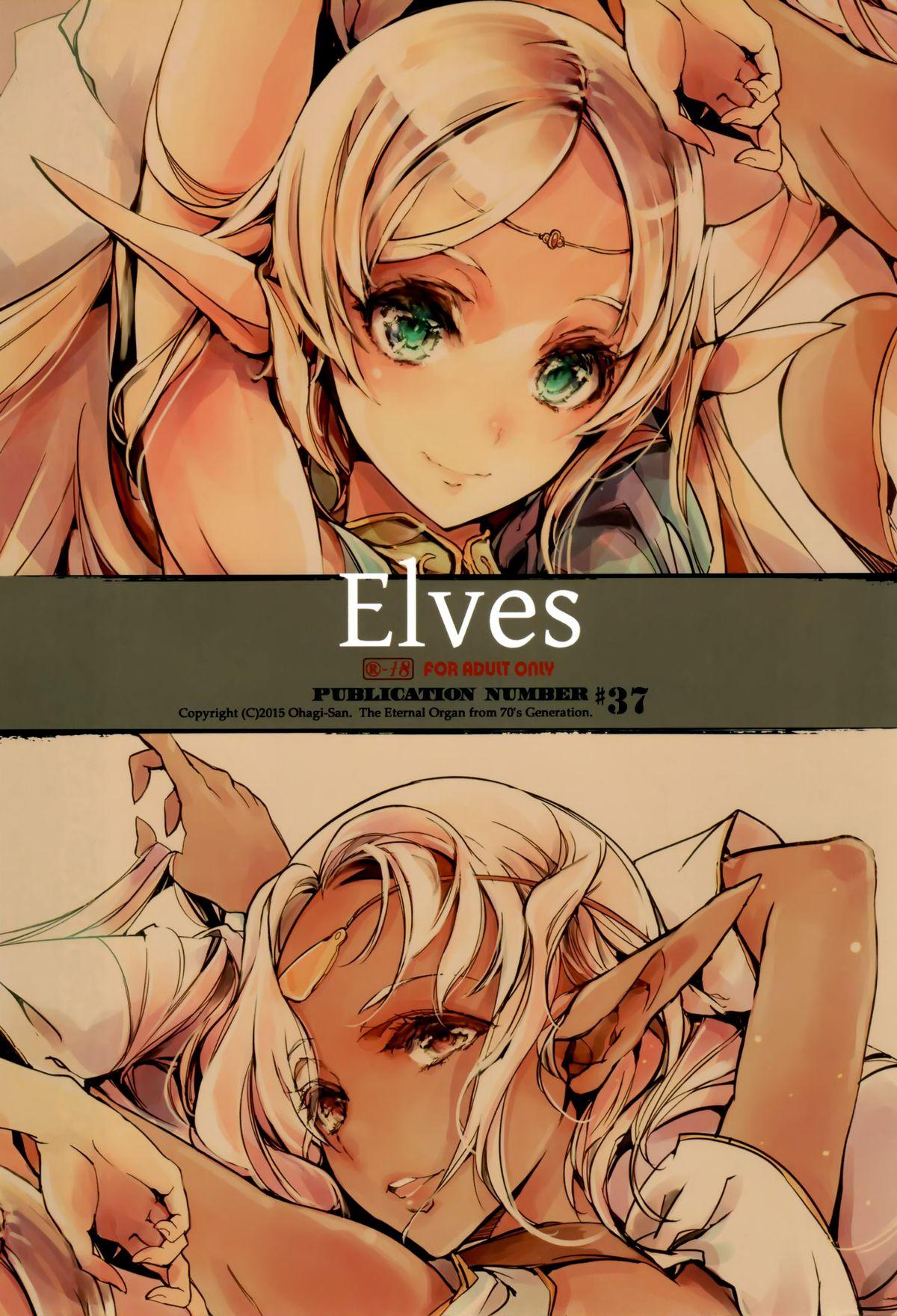The image depicts the cover of an adult-themed art book, titled "Elves," prominently displayed in the middle on a pewter-colored banner. The banner reads "Elves" in white text, "R-18 For Adults Only" in red, and "Publication Number 37" in black, with a copyright notice indicating "C. 2015." The cover is split horizontally into two different drawings of female elves. 

At the top, a young woman with large green eyes, pointed ears, and brown hair adorned with a silver chain around her forehead is shown. She is dressed in a sleeveless green tunic and appears to be raising her hands, although this is partially obscured in the image.

The bottom half features another female elf with long blonde hair. This elf also has pointed ears and seems to be in a reclining position, with her arms behind her head, similar to the arrangement of the top image. Both figures are depicted in a style reminiscent of anime, and neither is fully clothed within the visible frame of the cover. This detailed illustration hints at the adult nature of the book, emphasizing its R-18 rating. 

In the background, there are faint, indistinct forms that resemble other characters or elements, adding to the intricate artistic design meant to appeal to fans of anime-styled fantasy art.